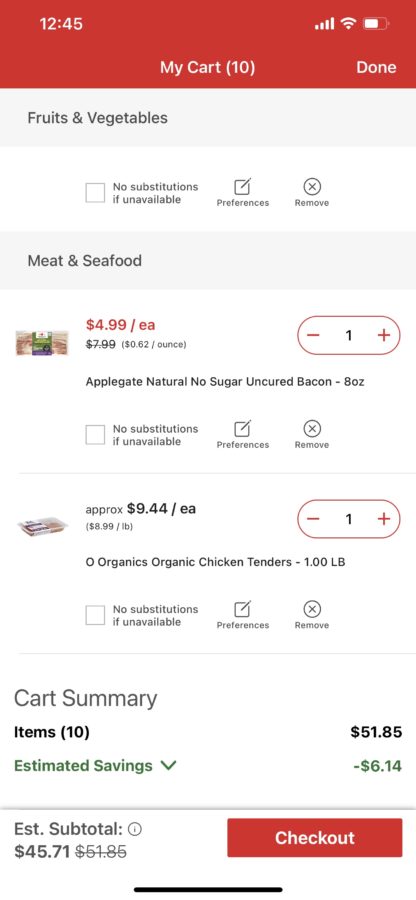The image is a detailed screenshot of a mobile phone displaying a shopping cart interface on a grocery website. At the very top, there is a prominent red banner featuring white text and icons. On the top left corner of the banner, the number "1245" is displayed, indicating the current time. In the center of the banner, the text "My Cart" is shown, followed by the number "10" in parentheses, which represents the number of items in the cart. On the top right, there are icons for signal strength, Wi-Fi connectivity, and battery life. To the right of the center text, there is a "Done" button in white.

Below the red banner, the background changes to white, with the black text "Fresh Fruits and Vegetables." Right under this section is an unchecked checkbox next to the text "No substitutions if unavailable." Accompanying this are two buttons labeled "Preferences" and "Remove."

Following this section, there are itemized listings with photos beginning with the category "Meat and Seafood." The first listed item is displayed with a photograph, accompanied by the price "$4.49 each" in red text. Below the price is the item description: "Applegate, Natural, No Sugar, Uncured Bacon." Adjacent to this description is an oval button with a "1" in the center, and "-" and "+" buttons on the left and right sides, respectively, for adjusting the quantity. Additional buttons for this item include "No substitutions if unavailable," "Preferences," and "Remove."

The second item listed is "Organic Chicken Tenders (one pound)," with an approximate price of "$9.44 each" above the description. This item also has the same quantity-adjusting oval button and the accompanying options for "No substitutions if unavailable," "Preferences," and "Remove."

Lower down, in black text, the headings "Cart Summary" and "Items (10)" are displayed. Below this, "Estimated Savings" is shown in green text with a downward-pointing arrow. To the right, the total amount for items is listed as "$51.85." The estimated savings of "-$6.614" is also shown in green. Below these totals, the text "Subtotal" appears, followed by "$45.71," and "$51.85" is struck through beside it.

At the bottom right corner, there is a red rectangular "Checkout" button with white text. Finally, a small black line runs across the center at the very bottom of the screen.